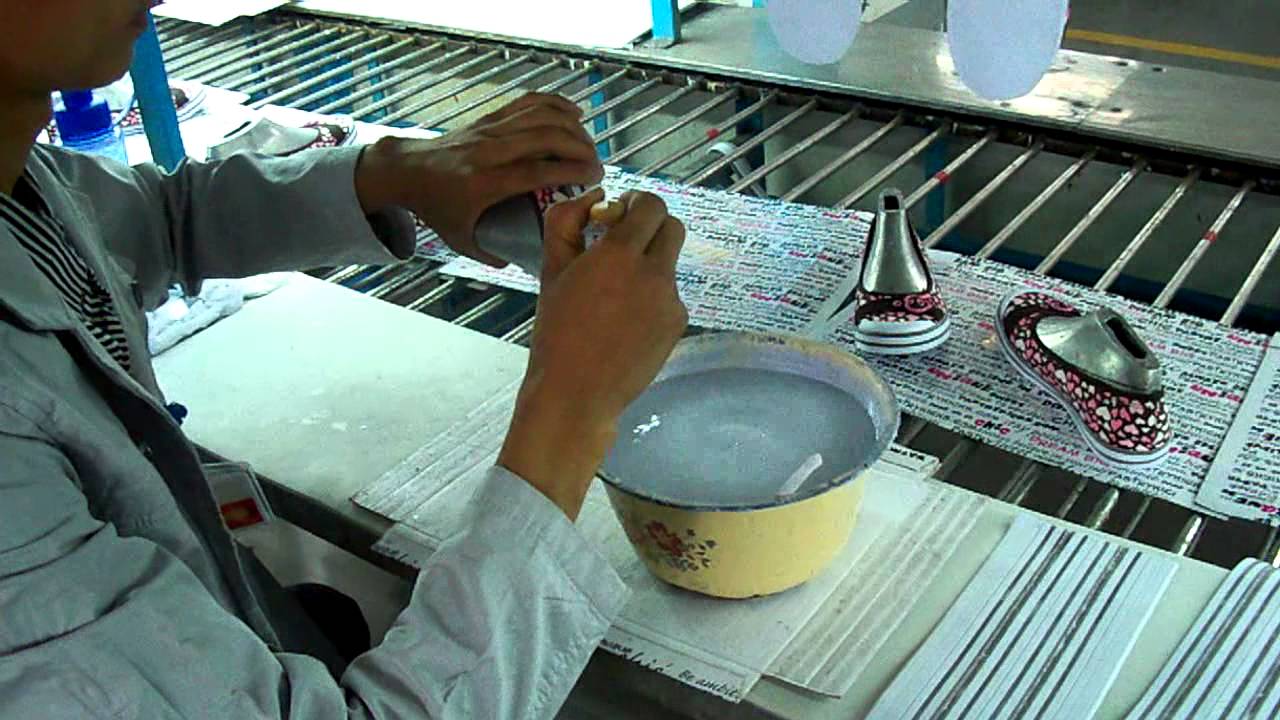In this detailed photograph, we find ourselves in an industrial setting featuring stainless steel tables with racks made of steel bars. Arranged on a narrow row of paper in the middle of these racks, we see children's shoes. These shoes, in various colors such as black, brown, and white, are adorned with pink hearts and feature little buckles. They are placed on stainless steel foot molds to maintain their shape. 

At the forefront of the image stands a man dressed in a long-sleeve white coat and a black-and-white striped shirt, with a name badge clipped to his coat. His face is partially obscured, but his chin and jawline are visible. He is engrossed in his work, holding a matching shoe over a bowl containing a clear liquid, possibly resin or water. The bowl, ceramic with a yellow floral design on the outside and white on the inside, is placed on a counter covered with mats and towels. To the left of the man, atop the racks, more of these decorated children's shoes are neatly arranged, completing this intricate scene.